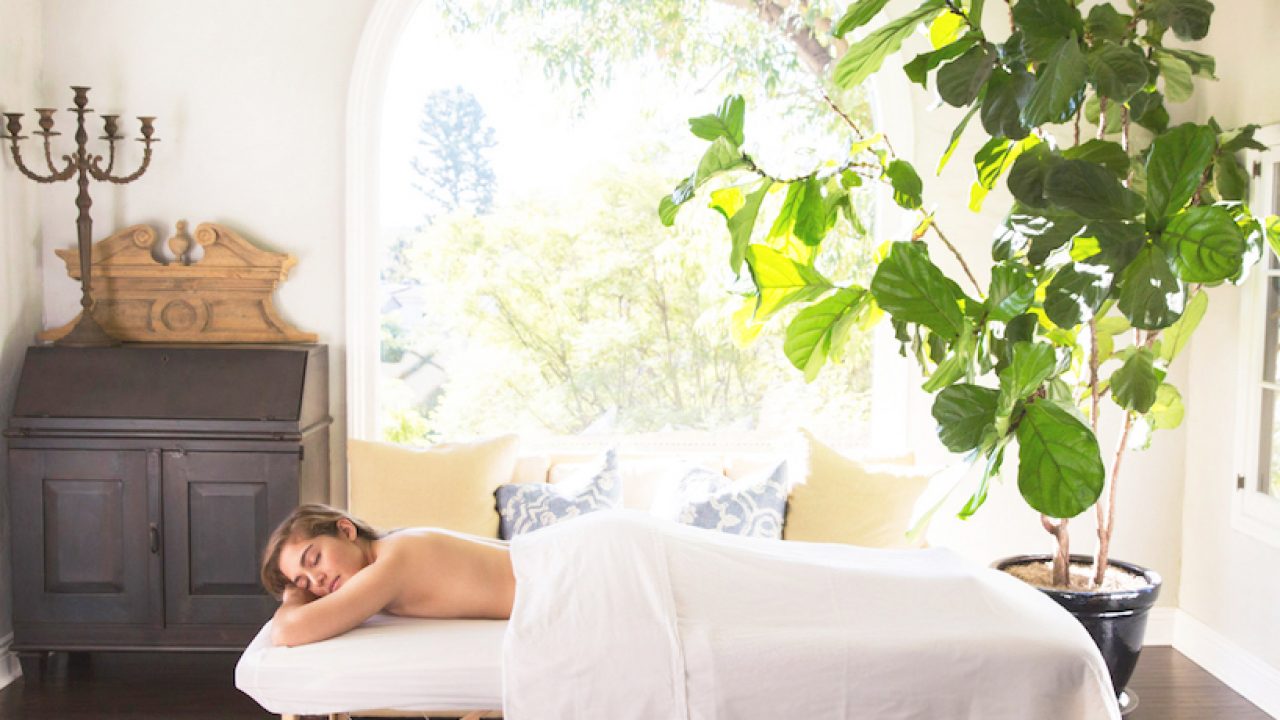The image captures a serene spa setting with a young woman lying face down on a white-covered massage table. She has light brown hair and her head rests on her crossed forearms, with her eyes closed, exuding a sense of deep relaxation. A white sheet drapes over her lower body, leaving her back exposed. The room is softly illuminated by daylight streaming through an arched window in the background, although the view is obscured by bright sunlight. To the right of the massage table stands a tall potted plant with lush, green leaves reaching towards the ceiling, adding a touch of nature to the calm atmosphere. On the left side, there's a dark brown wooden stand, topped with a candelabra, providing a rustic accent to the room. The setting also includes a cozy sofa adorned with blue pillows and a couple of beige ones, enhancing the inviting ambiance. A white wooden door is visible to the right, completing this tranquil, spa-like oasis.